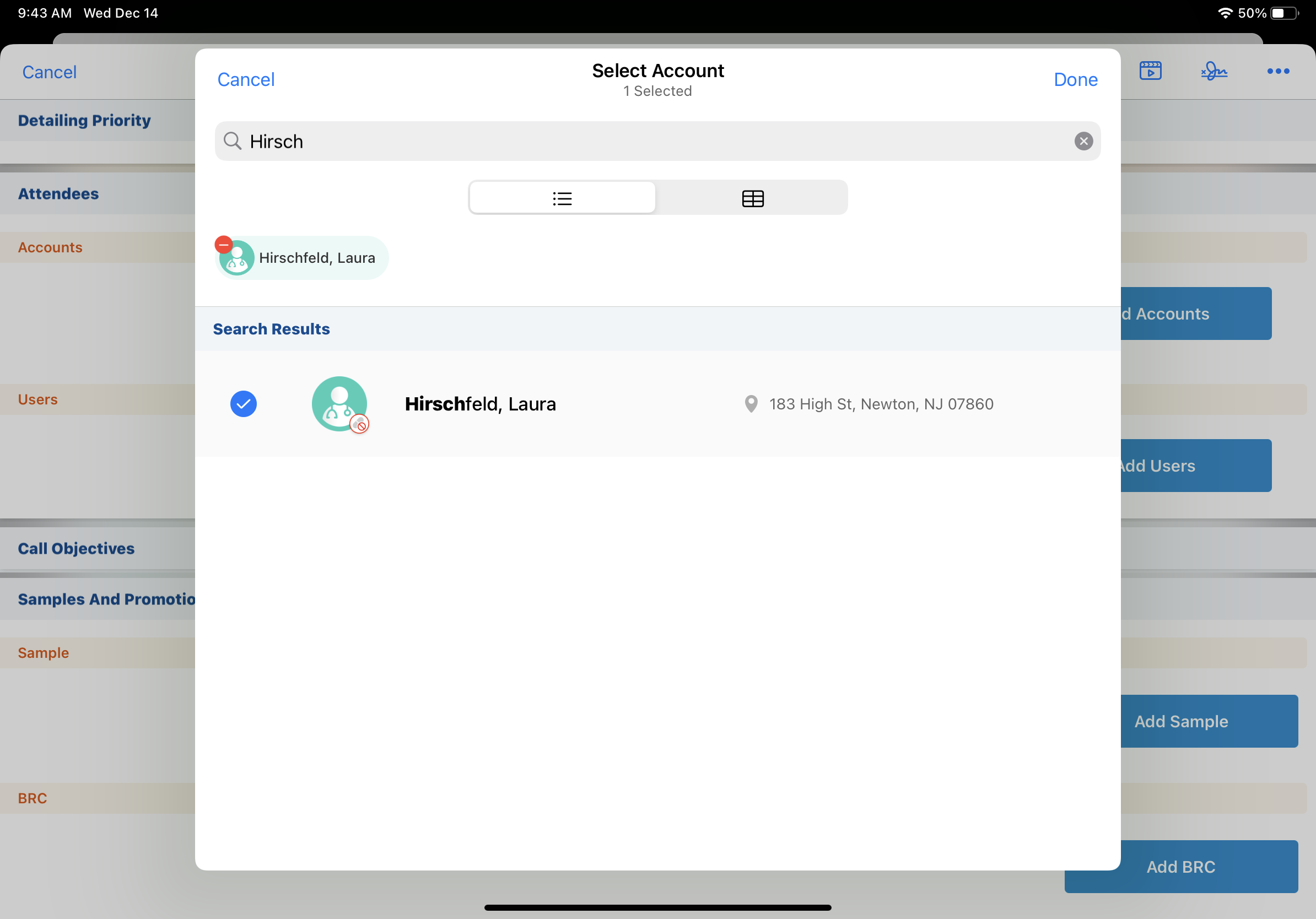The image depicts a screenshot of a website viewed on a mobile device. The thin black status bar at the top displays the date and time: "9:43 a.m. Wednesday December 14th." On the right side of this bar, there are full Wi-Fi signal bars and a battery icon showing 50% charge.

An information box pops up in the center of the screen with the heading "Select Account - 1 Selected." The top-left corner of the box features a "Cancel" button in blue, while the top-right corner showcases a "Done" button, also in blue. Below the heading, there is a light gray search box with the text "Hirsch" entered into it.

The middle section of the pop-up box has two viewing options: a list view (selected) and an icon view. Listed next is "Hirschfield, Laura" in a mint green highlight, indicating the selected account. Below this, the search results display with a blue checkmark next to "Hirschfield, Laura 183 High Street, Newton, New Jersey 07860," along with a location pin icon.

Behind the pop-up box, the underlying webpage is partially visible. On the left side of this page, there's a "Cancel" option. Below it, several menu items are listed: "Detailing Priority," "Attendees," "Accounts," "Users," "Call Objectives," "Samples," and "Promotions." Near the bottom of this partial view, there are sections labeled "Sample" and "BRC."

This detailed description captures the elements and layout present in the image.